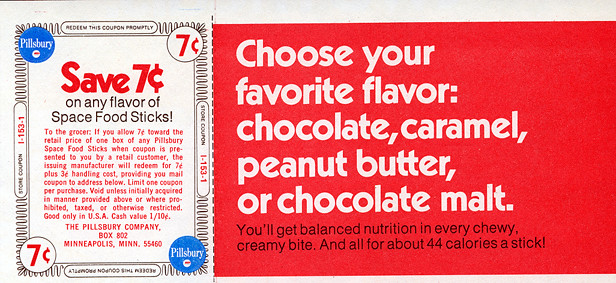This vintage advertisement features a classic Pillsbury promotion. On the left side, the ad is printed on white paper and includes a small blue circle in the top left corner displaying the Pillsbury logo. The main text on this side announces a special offer: 'Save seven cents on any flavor of Space Food Sticks.' On the right side, a prominent red backdrop draws attention with bold, white letters encouraging consumers to 'Choose your favorite flavor: chocolate, caramel, peanut butter, or chocolate malt.' Below this, smaller black text highlights the product's nutritional benefit, stating, 'You'll get balanced nutrition in every chewy, creamy bite. And all for about 44 calories a stick.' The combination of striking visuals and enticing text aims to make an appealing call to action for prospective buyers.